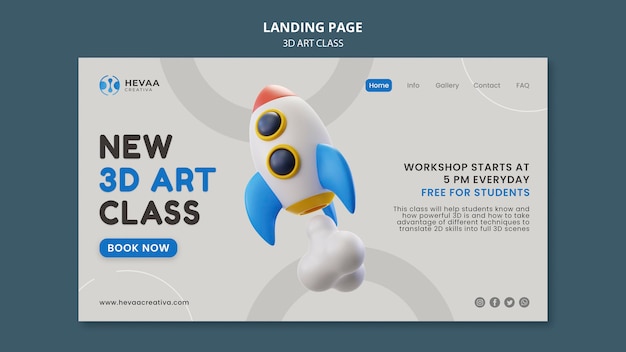This visually engaging advertisement appears to be either a website banner or magazine ad promoting a 3D art class. The background is divided into four screens with a central gray rectangular panel. Above this central panel, there is a green background that transitions into white, adorned with a bold "Landing Page" title in 3D, followed by "3D Art Class" in white text beneath it.

At the heart of the image, a whimsically designed 3D rocket—colored in red, white, yellow, black, and blue—takes off diagonally towards the upper left corner, leaving a trail of white smoke. Positioned at the top left is a circular blue icon, accompanied by the text "HEVAA" in black. Directly underneath this, the word "NEW" is prominently displayed in large, bold black letters.

Central to the ad, the words "3D Art" appear in blue text, followed by "Class" in large black letters. Below this, a blue oval button with white text invites viewers to "Book Now," while the lower left corner features a black URL for further information.

In the upper right, a blue button with white text labeled "Home" is visible, along with three black-titled sections: "Info," "Gallery," "Contact," and "FAQ." Just beneath these buttons, informative text in black announces that the "Workshop starts at 5 p.m. every day," and in blue, it highlights that it is "Free for Students." Further down, a paragraph elaborates on the class objectives and instructional approach.

The bottom right corner showcases four social media icons—Instagram, Facebook, Twitter, and an unidentified gray and white icon—completing this comprehensive and eye-catching design.